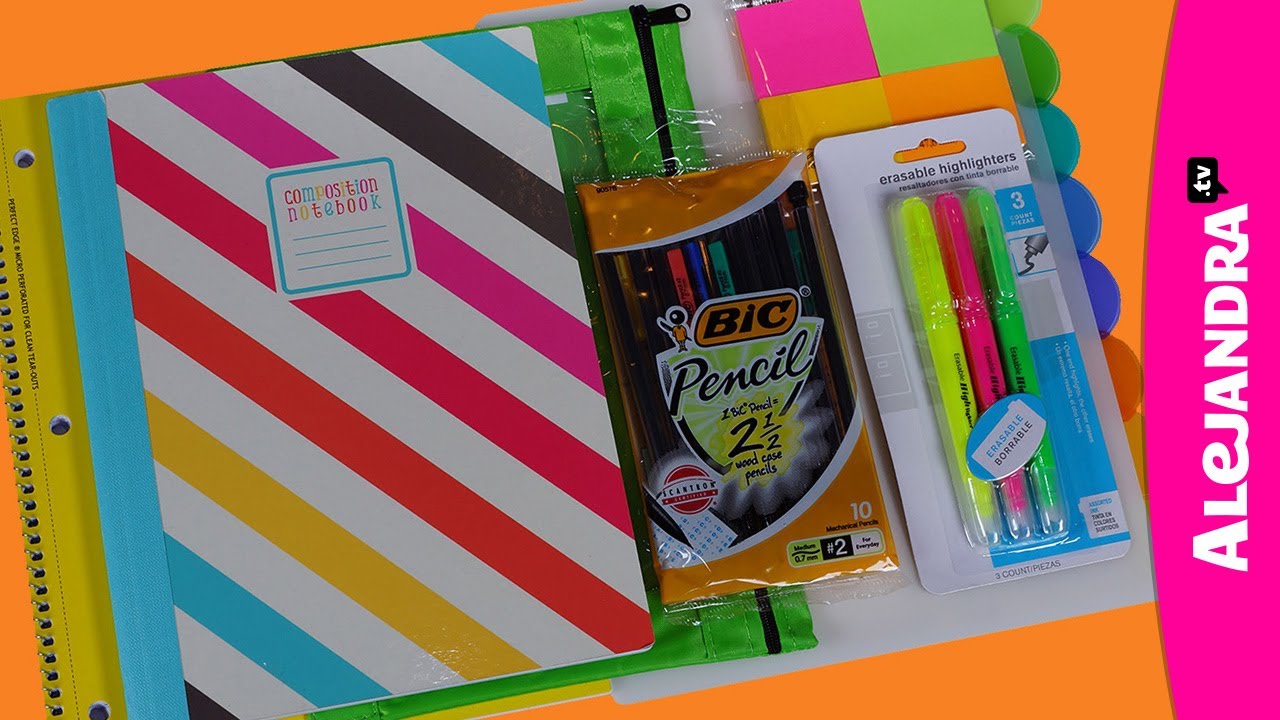The image features a carefully arranged assortment of back-to-school supplies set against a colorful background. Central to the composition is a vibrant composition notebook with diagonal rainbow-colored stripes, bound with a blue edge. This notebook is placed on top of a clear green pencil pouch and a yellow notebook, partially obscuring its details. To the right, there is a sealed pack of ten Bic mechanical pencils. Adjacent to the pencils, three erasable highlighters—yellow, pink, and bright lime green—are neatly packaged and positioned. Behind these items, a binder with section tabs and an array of colorful sticky notes (pink, green, yellow, and orange) is visible. Completing the scene, the phrase "Alejandra TV" is prominently displayed on a pink nameplate or binder holder, with "Alejandra" in white text and "TV" in a black speech bubble on the right. The image perfectly captures a well-organized back-to-school kit, combining functionality with a splash of color.